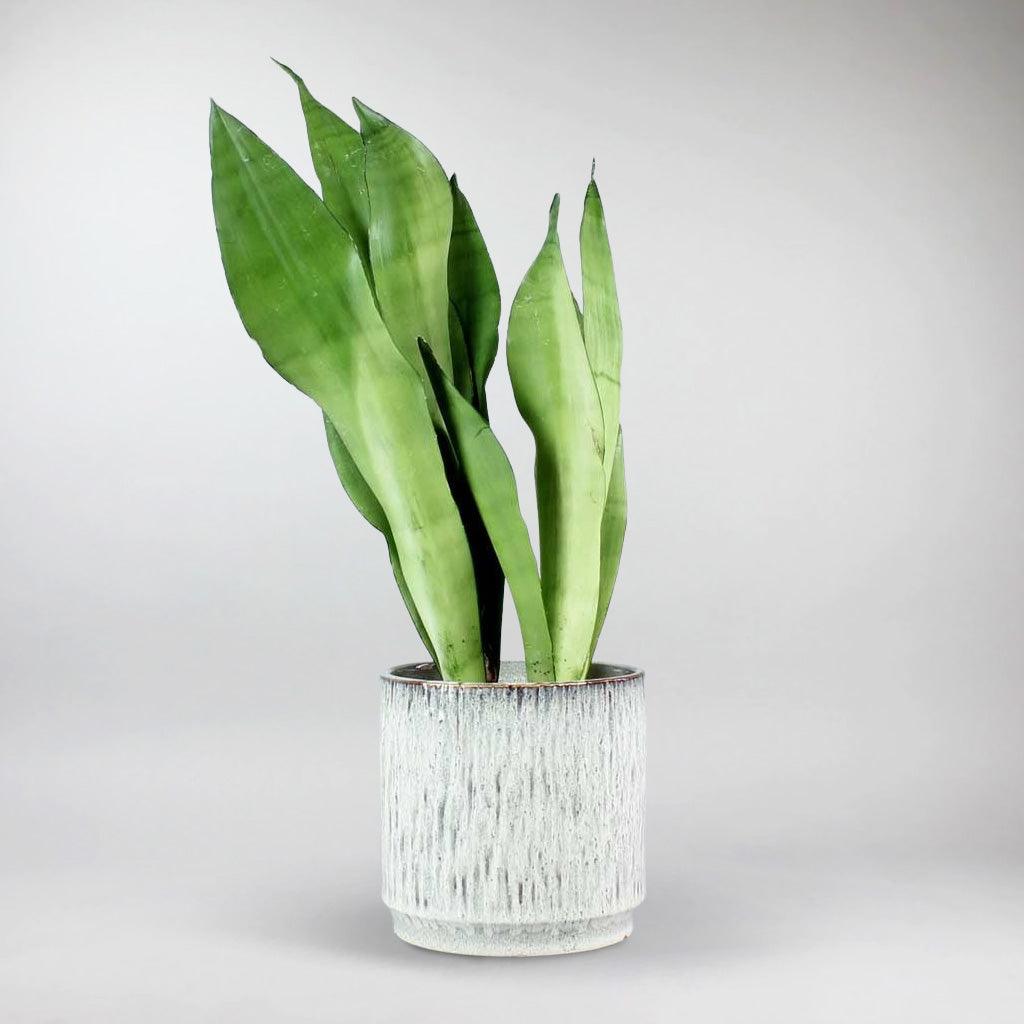The image depicts a minimalistic and modern plant product photo, with a focus on a planter placed centrally on a white surface against a light gray to slightly darker gradient background. The planter, which has a cylindrical and cup-like shape, appears to be ceramic and features a distressed white finish with vertical black and gray streaks, adding an aged and textured appearance. Emerging from the planter are approximately 10 long, green leaves. These dagger-shaped leaves rise sharply, becoming progressively darker and more mature at the tips, with some clustered on the left side and others on the right. The overall simplicity and clean design highlight the planter and the growing plant as the main subjects of the image.